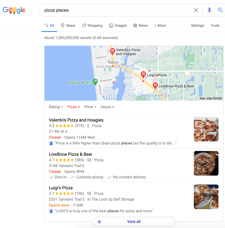This image, set against a white background, features a blurred Google search results page. In the upper left corner, the Google logo is present, with the "OO" replaced by Christmas lights in red and yellow. The map displayed within the search results shows water to the west and land to the east, with three red pins and one green pin marking locations.

Below the map, three search result listings are visible. The first listing shows what appears to be "pizza and hoagies" with a 4.3-star rating and an accompanying photo of a pizza on the right. The second listing mentions "pizza and beer," though the details are unclear. The third listing prominently displays "Luigi's Pizza" in bold black text with a 4.7-star review and a photo of the restaurant's interior to the right.